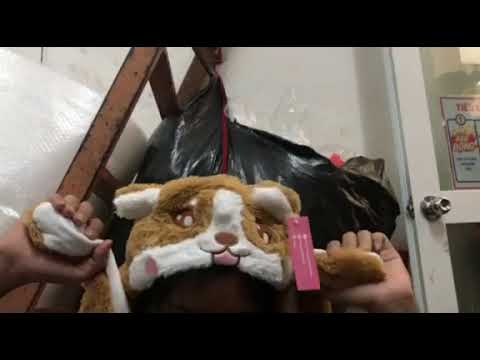This photograph depicts the interior of a room with white walls accented by two horizontal black strips at the top and bottom. Central to the image is the top portion of a person’s head adorned with a whimsical hat resembling a stuffed animal. The hat, designed like a dog, features brown fur with white accents on the inner ears, face, and paws, coupled with a pink tongue, brown nose, and brown-and-white eyes. The person’s peach-colored hands are visible, holding the hat’s paws. Behind this individual, a brown ladder leans against the wall, to which a large black garbage bag with red string is attached, appearing to be stuffed with indistinguishable items. To the right side of the composition, there is a white door with a silver handle and glass panes, contributing to the room's overall sparse yet curious aesthetic.